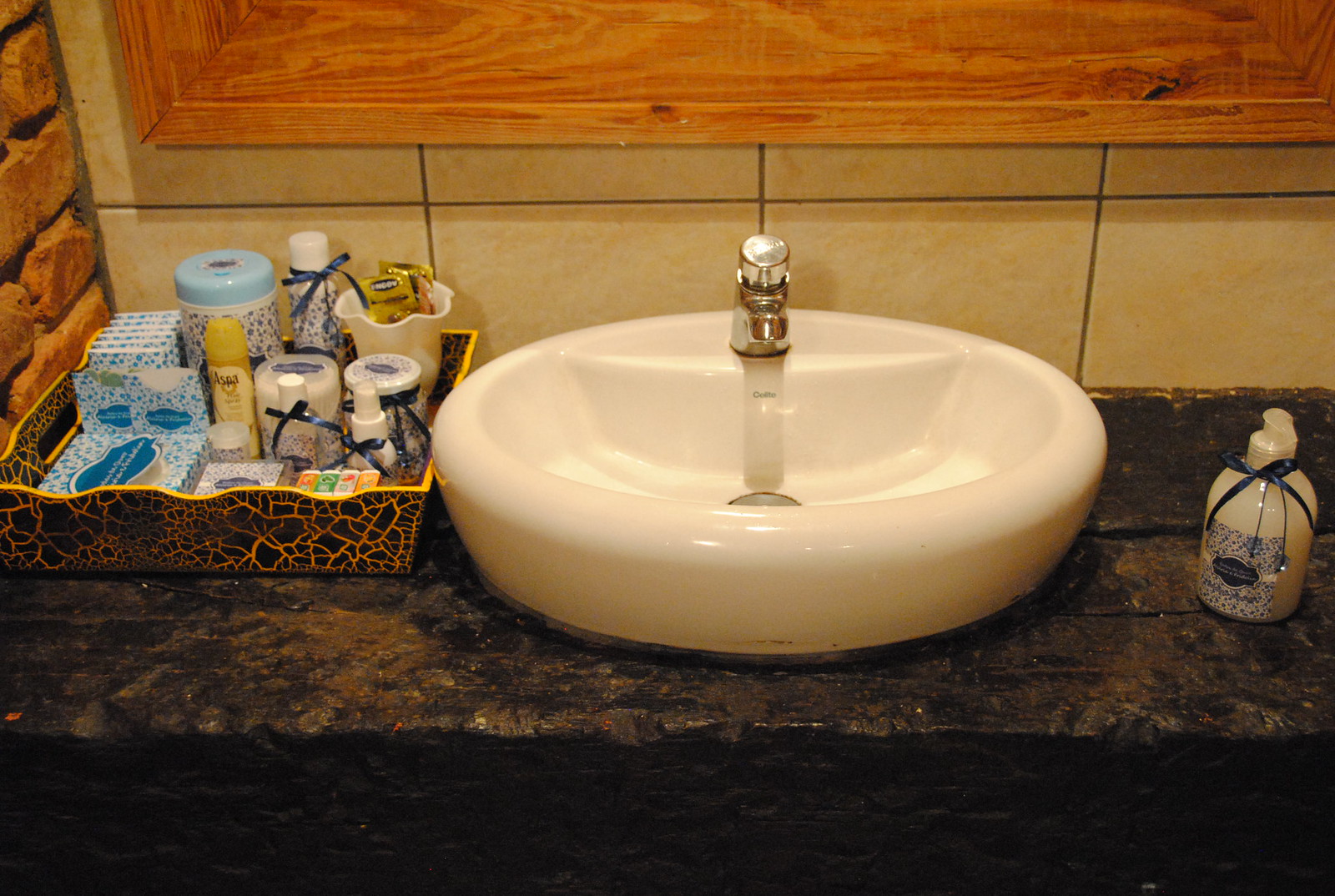This photograph showcases a detailed scene centered around a thick, black countertop that features a myriad of bumps and cracks, some of which have hints of brown. Prominently situated in the middle of the countertop is a pristine white sink, adorned with a sleek silver faucet and a minor brown mark on its surface. The sink also reveals a glimpse of its silver drain at the bottom. Positioned to the right of the sink, a bottle filled with white liquid stands with a pump on top, decorated with a blue ribbon and a label that displays blue writing. To the left of the sink, a yellow and black basket brims with various small bottles, each adorned with tiny ribbons. Above the sink, a brown board begins to form the backdrop for a mirror, while immediately to the left of this setup, a section of brown brick accentuates the overall rustic aesthetic of the scene.